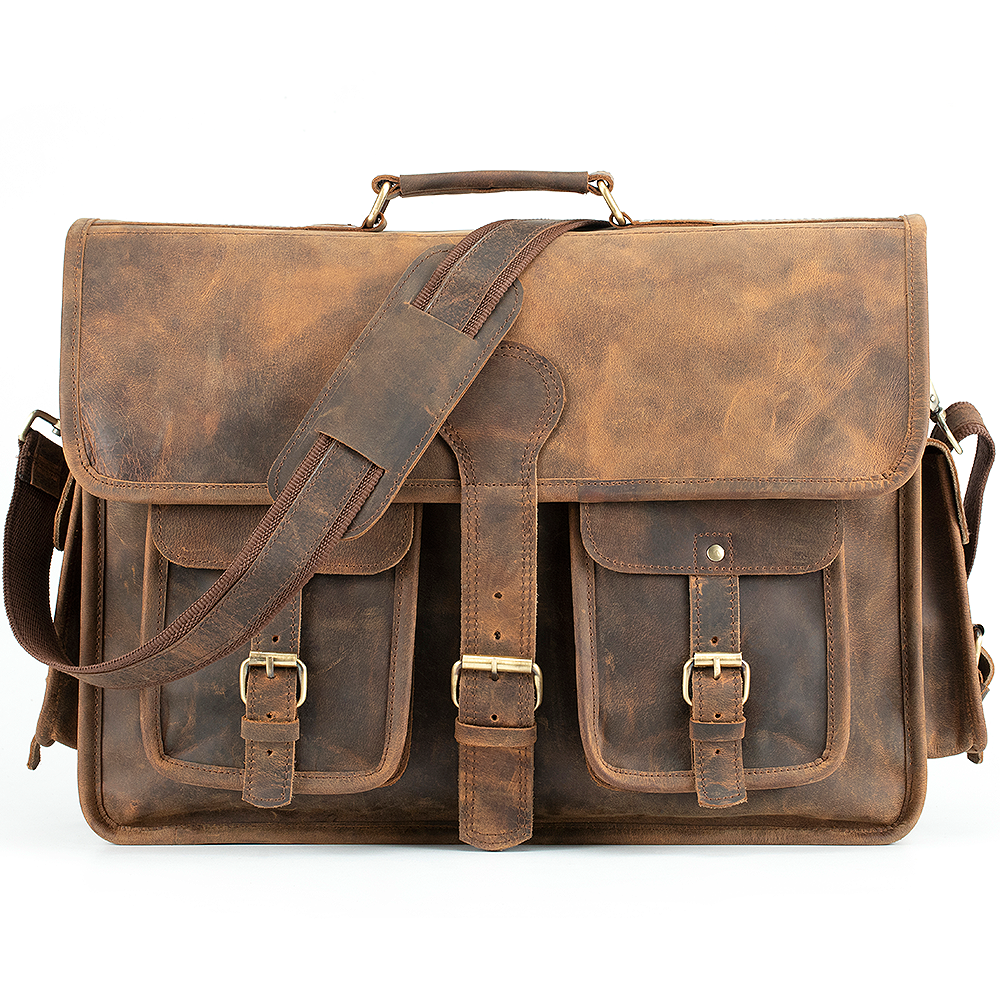This image shows a vintage-style, distressed brown leather messenger bag. The bag features a worn-in appearance, reminiscent of those seen in historical photographs of mail carriers or travelers. It has a top handle attached by silver clasps and a padded shoulder strap for comfortable cross-body wear. The bag boasts multiple pockets, with two on the sides and two on the front, all secured by brass or nickel-plated buckles. The main flap also buckles down to secure the contents inside. This spacious bag is ideal for carrying a laptop, important papers, school supplies, or work essentials, making it both a functional and stylish accessory.